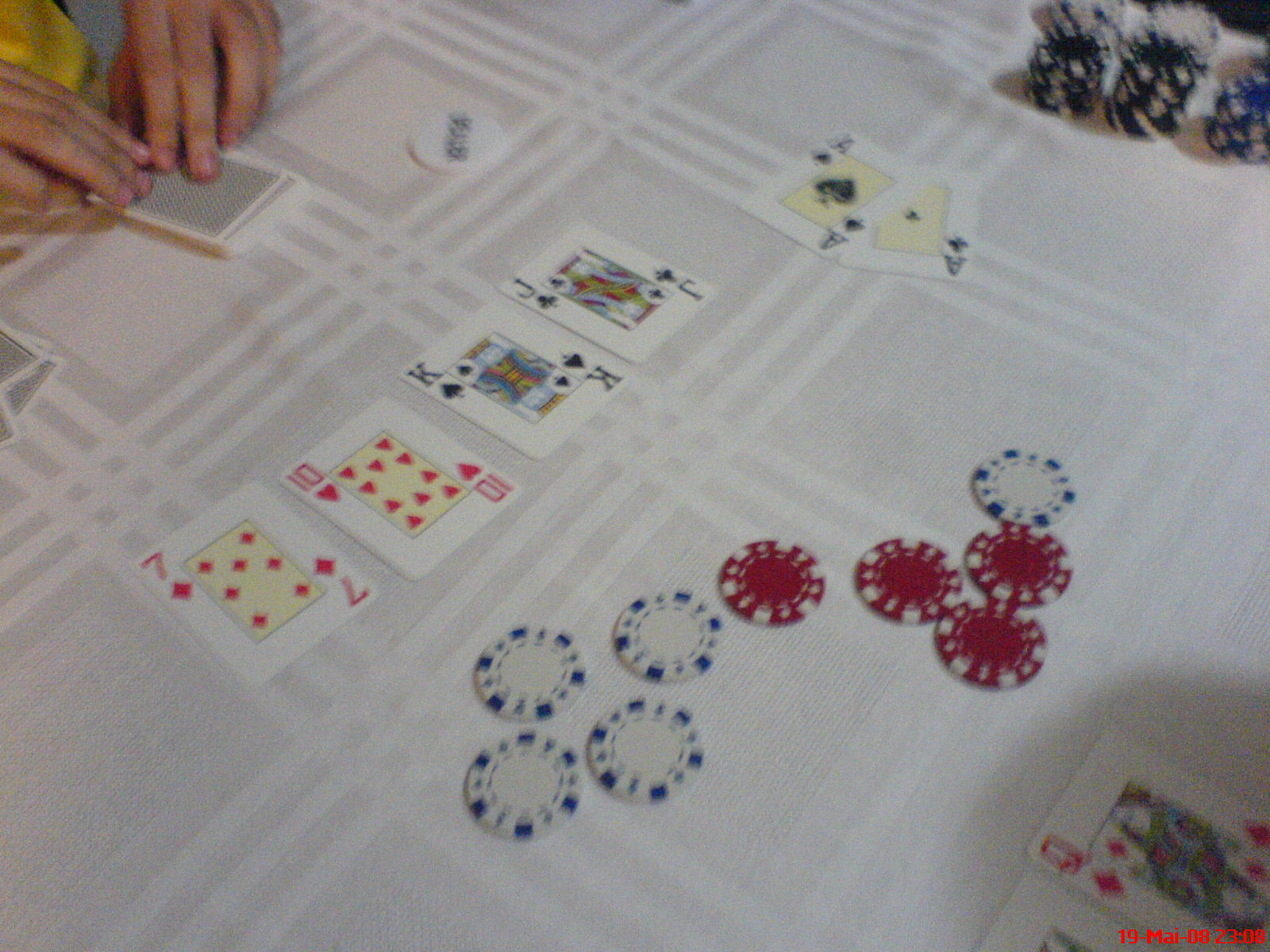In this indoor photograph, a game of poker is in progress on a table adorned with a white tablecloth featuring a lined pattern. The scene is filled with various playing cards laid out on the table, including a seven of diamonds, a ten of hearts, a king of clubs, an ace of spades, an ace of clubs, and a queen of diamonds, each displaying their distinctive red, black, and white designs. Scattered around the cards are several poker chips, contributing to the lively atmosphere. Five blue and white poker chips and four red and white plastic poker chips are prominently featured. Towards the end of the table, a neat stack of black and white poker chips forms two rows, while a smaller arrangement of blue and white poker chips is piled on top of each other. A pair of white hands, caught in the action of dealing cards, adds a dynamic human element to the composition.